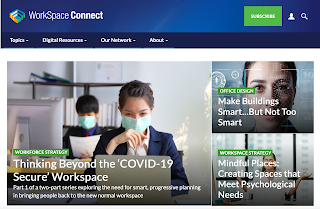The image displays a screenshot of a webpage, organized into three distinct frames. The top horizontal frame has a blue background featuring a logo resembling a shield on the left side. To the right of the logo, written in white text, are the words "Workspace Connect." On the far right side of this blue frame, there is a green button, alongside icons of a person and a magnifying glass, which represent user profile and search functionalities respectively.

The main content frame below is split into two sections. On the left side, the larger section showcases a high-resolution image of two individuals dressed in dark blue suits, both wearing light blue face masks. Subtly overlaid in white text beneath this image are the words “Thinking Beyond – Creating a COVID-19 Secure Workspace.” 

On the right side of the main content frame, two smaller images are stacked vertically, completing the page’s visual layout. The thoughtful design and imagery underscore the theme of maintaining safe and productive work environments in a post-pandemic world.